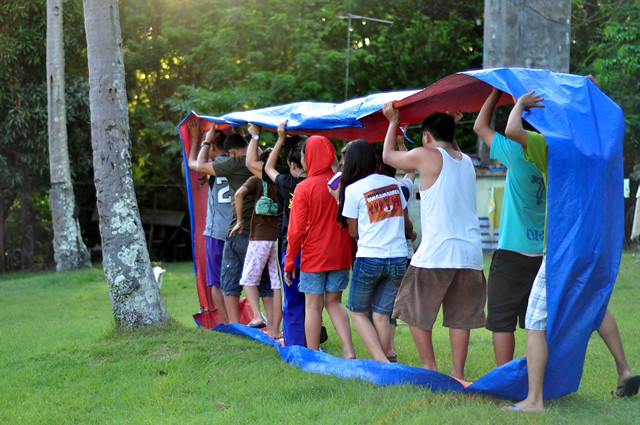In this outdoor photograph, a large grassy field with well-trimmed, bright green grass is bordered by a lush forest of various trees showcasing dense, green foliage. Several thick, gray tree trunks emerge from the grass but are cut off at the top of the image. Near the forest's edge, a partially visible streetlight or lamp post stands. A group of eight to ten teenagers, dressed casually in shorts, t-shirts, tank tops, and some jackets, are engaged in what appears to be a team-building exercise. They are positioned in a single line, each person holding a long, circular piece of vinyl tarp, colored blue and red. The tarp stretches from their feet and is held overhead, creating an archway as they move forward together, suggesting a collaborative and fun activity.